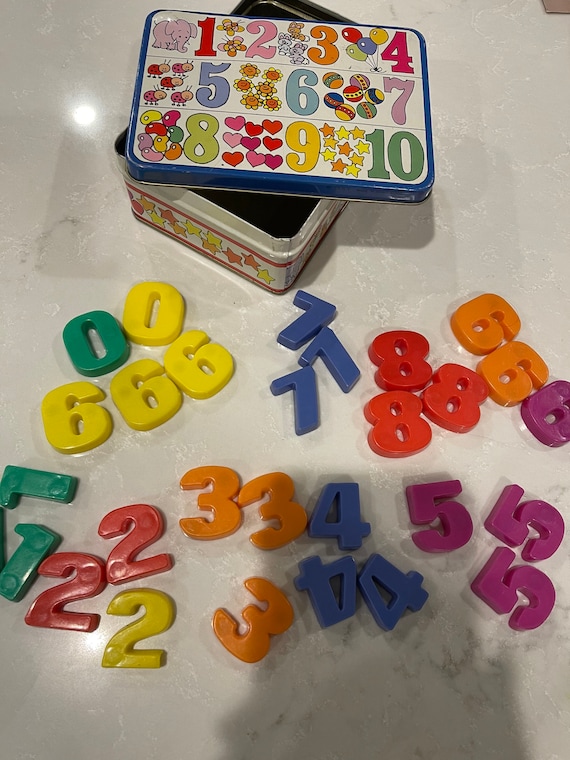The photograph depicts a nostalgic, old-time child's educational playset. At the center of the image is a slightly open, vintage metal tin with its lid resting beside it. The tin, positioned on a white, possibly marble table, is adorned with illustrations of hearts, flowers, and balls, and is decorated with colorful numbers from 1 to 10. Each number on the tin is paired with playful images like elephants and balloons that increase in quantity with the numbers.

In front of the tin, a collection of brightly colored, hard plastic magnetic numbers (ranging from 0 to 8) are scattered across the surface. These numbers, in shades of red, blue, yellow, orange, green, and purple, are grouped in clusters but not perfectly ordered. The playful hues and arrangement of the numbers, featuring multiple instances of each digit, add to the nostalgic, cheerful vibe of the scene, reminiscent of a child's learning toy from the 1980s.